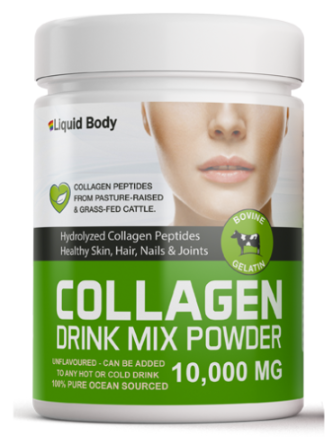The image depicts a white plastic container with a white lid, resembling a small tub, labeled with various colorful and detailed graphics. At the top of the label, the text "Liquid Body" is prominently displayed, followed by a small rainbow stripe featuring red, yellow, and blue colors. Just below this, in larger text, it reads, "Collagen Peptides from Pasture-Raised and Grass-Fed Cattle." Adjacent to this text is a distinctive green heart symbol, which incorporates a white leaf shape as a part of its design.

The label also features an image of a woman’s face, but only from the cheekbones down to the chin, highlighting her lips and ears. Positioned beneath this image is a black band with the text "Hydrolyzed Collagen Peptides," and additional benefits listed as "Healthy Skin, Hair, Nails, and Joints." Embedded within this black band, there is a green circle containing an illustration of a black and white cow, along with the terms "Bovine Gelatin."

The lower part of the label has a green background with white text stating, "Collagen Drink Mix Powder." It specifies that the product is unflavored and can be added to any hot or cold drink, emphasizing its purity and ocean-sourced ingredients at "100% Pure Ocean Sourced" in white text. A finer detail at the bottom right indicates that the product contains "10,000 milligrams," written in a combination of white and yellowish text.